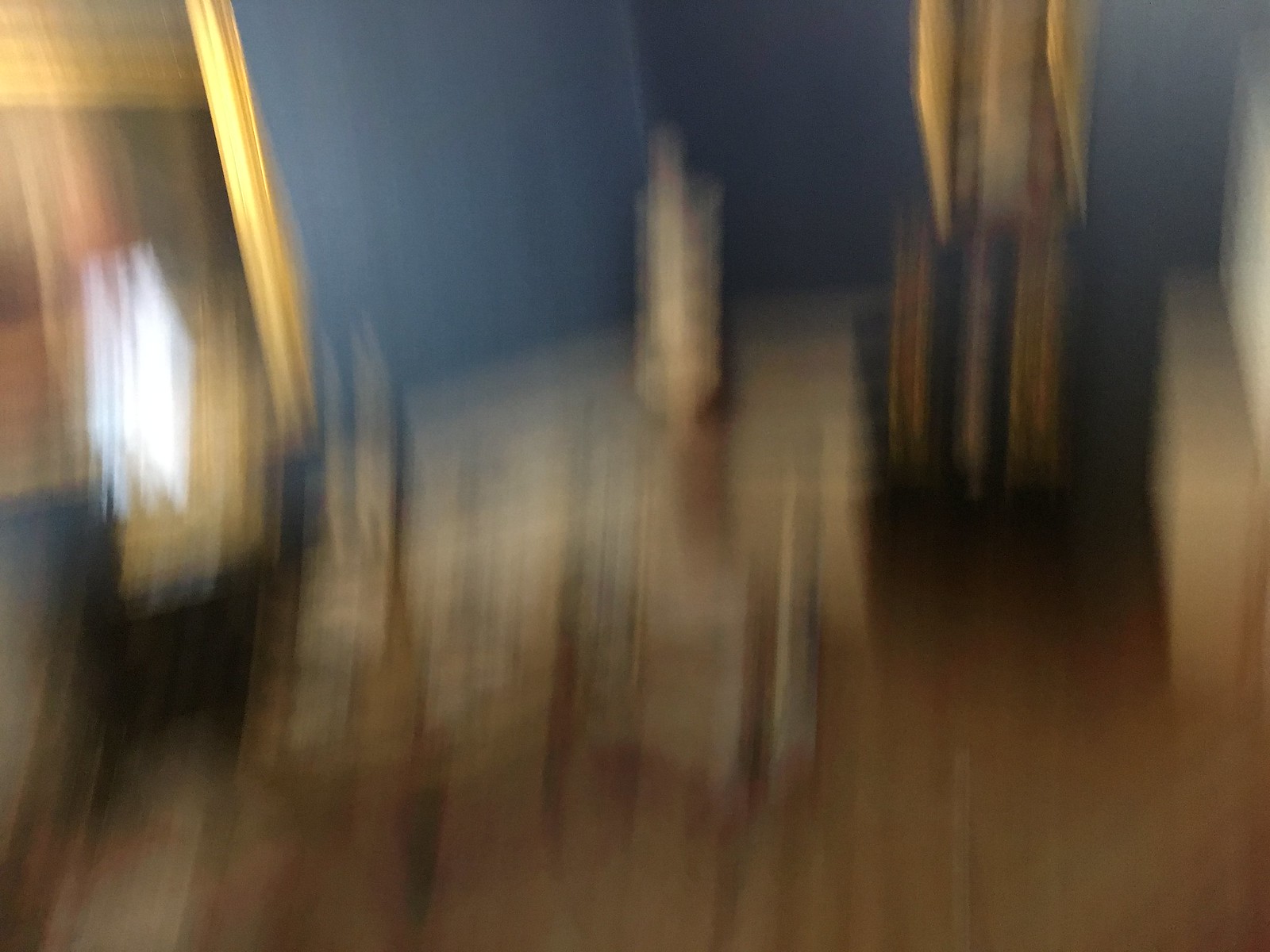The image is a horizontally oriented, extremely blurry photograph, likely taken indoors with noticeable motion blur. Dominant colors within the image include dark blue, gold, white, brown, and gray. The left side of the photo features what appears to be a shiny, gold-framed object, which could be a mirror or a painting. The walls in the background are a muted grayish-blue, suggesting an indoor setting such as a house or restaurant. A possible figure or object, white in color, occupies the center, while the right side features a gold and black item. Two cube-like, white objects are barely visible at the far right edge. The flooring is light tan wood, and there might be light-colored, possibly beige tables, along with some lights visible on the left.